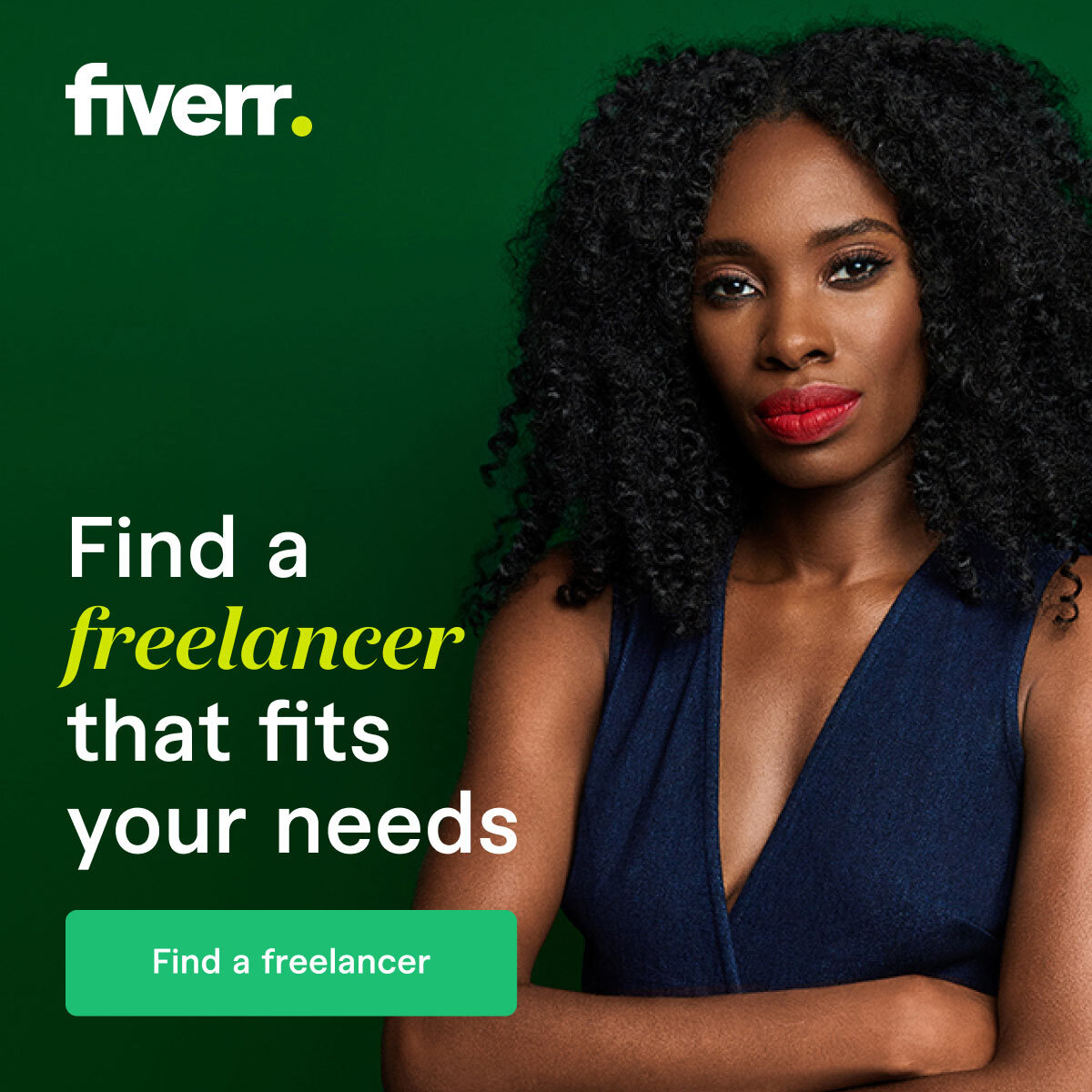The promotional image for Fiverr features a square design with a dark green background. Prominently placed in the top left corner is the Fiverr logo, written in white text with "Fiverr." completed with a distinctive yellow dot. On the right side of the image stands a young Black woman in her 20s or 30s. She has shoulder-length, curly black hair and brown skin. She is dressed in a navy blue vest over a white top. The left side of the image contains the text "Find a freelancer that fits your needs," highlighting the key message of the advertisement. Below this text is a green button with the call-to-action "Find a freelancer" written in white text. This image serves as an advertisement for Fiverr, emphasizing their freelance services.